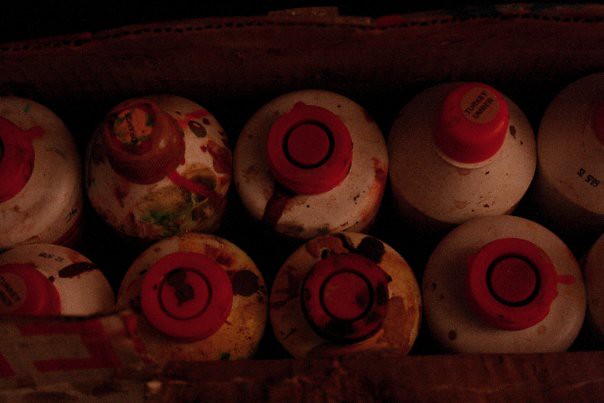This overhead photograph captures a cardboard box containing ten paint canisters, viewed from above. The box, made of corrugated cardboard, appears old and stained, with visible discolorations around its edges. Inside the box are two rows of paint bottles; the top row holds five canisters, while the bottom row contains four, with the first bottle of the bottom row partially visible.

Each bottle is round and fat, with small red caps. The bottles themselves are predominantly white but are heavily covered in paint splatters of various colors, including black, red, yellow, and some hints of green. A few of the bottles have stickers or labels; one notable label on the top of a cap reads "turkey umber" in black letters, while others have illegible black text.

A piece of cardboard, cut across the top, partially covers the view from above, allowing a peek into the box's contents. The repeated theme of red-capped, paint-splattered white bottles, and the overall dark tone of the image, suggest a well-used and perhaps neglected assortment of artist paints. One cap even appears sealed with melted wax, indicating careful preservation of its contents. Despite the chaotic paint stains, the arrangement of the bottles in their old, stained cardboard box provides a glimpse into an artist's messy yet colorful world.